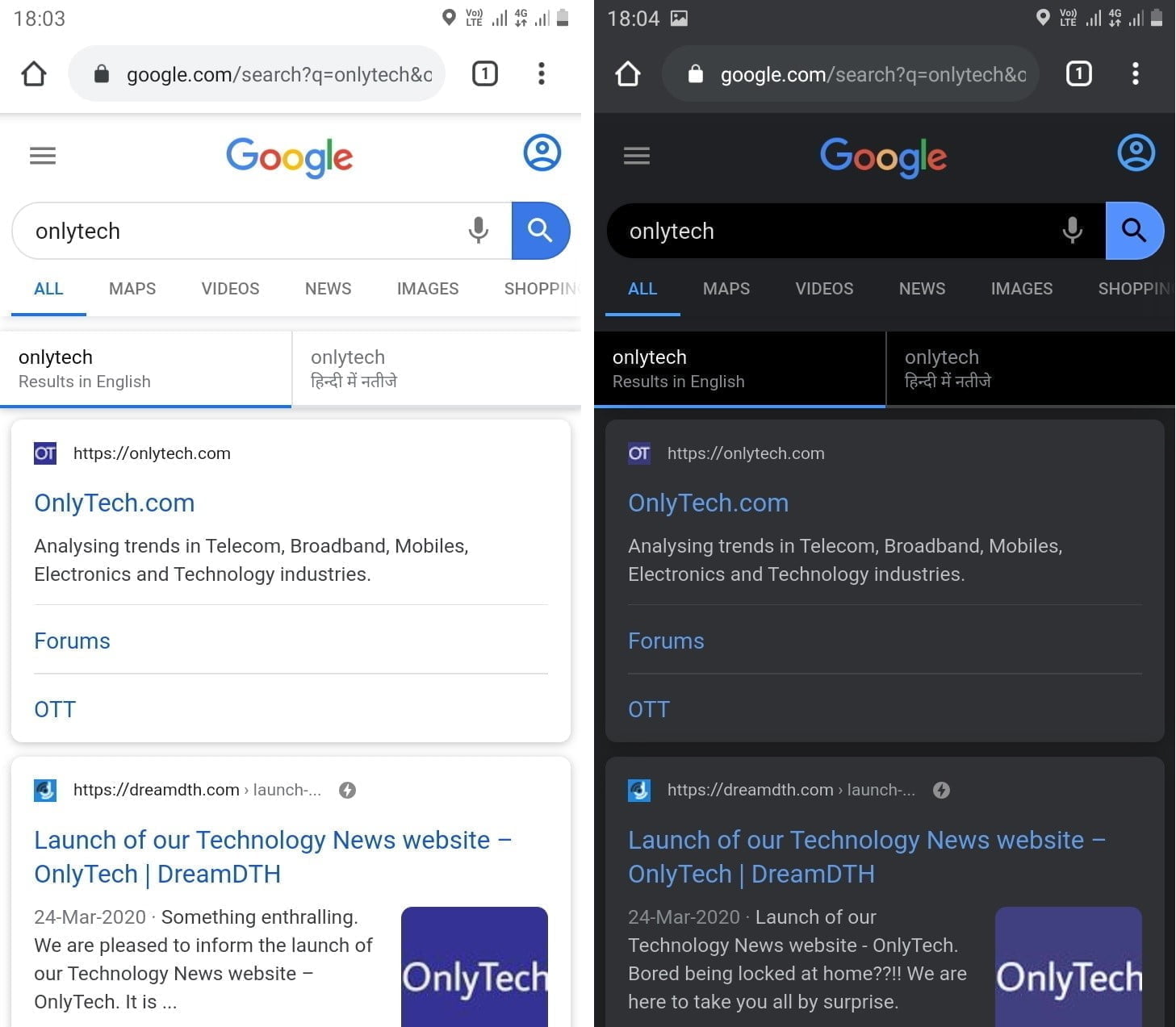The image features two vertical screenshots placed side by side, each showcasing the same webpage but with different background color settings. The left screenshot has a white background, displaying the time as 18:03 in the upper left-hand corner and a 20% battery level in the upper right-hand corner. The right screenshot features a black background, with the time changed to 18:04 and the battery level remaining at 20%.

Both columns display a Google search page with the query "Only Tech" entered, and each has one tab open. The search results are identical in both screenshots, starting with an underlined "Only Tech," followed by "Only Tech results in English" also underlined. The first search result is a live link to "onlytech.com," followed by live links to "Forums" and "OTT". The next URL is a title that reads "Launch of our technology news website, Only Tech." At the bottom right-hand corner of both screenshots, the page shows "Only Tech" prominently in the background.

This image highlights the choice between a light mode and dark mode for viewing the same content, showcasing user preference flexibility. The describer personally prefers the white background for better readability, while finding the black background difficult to read.